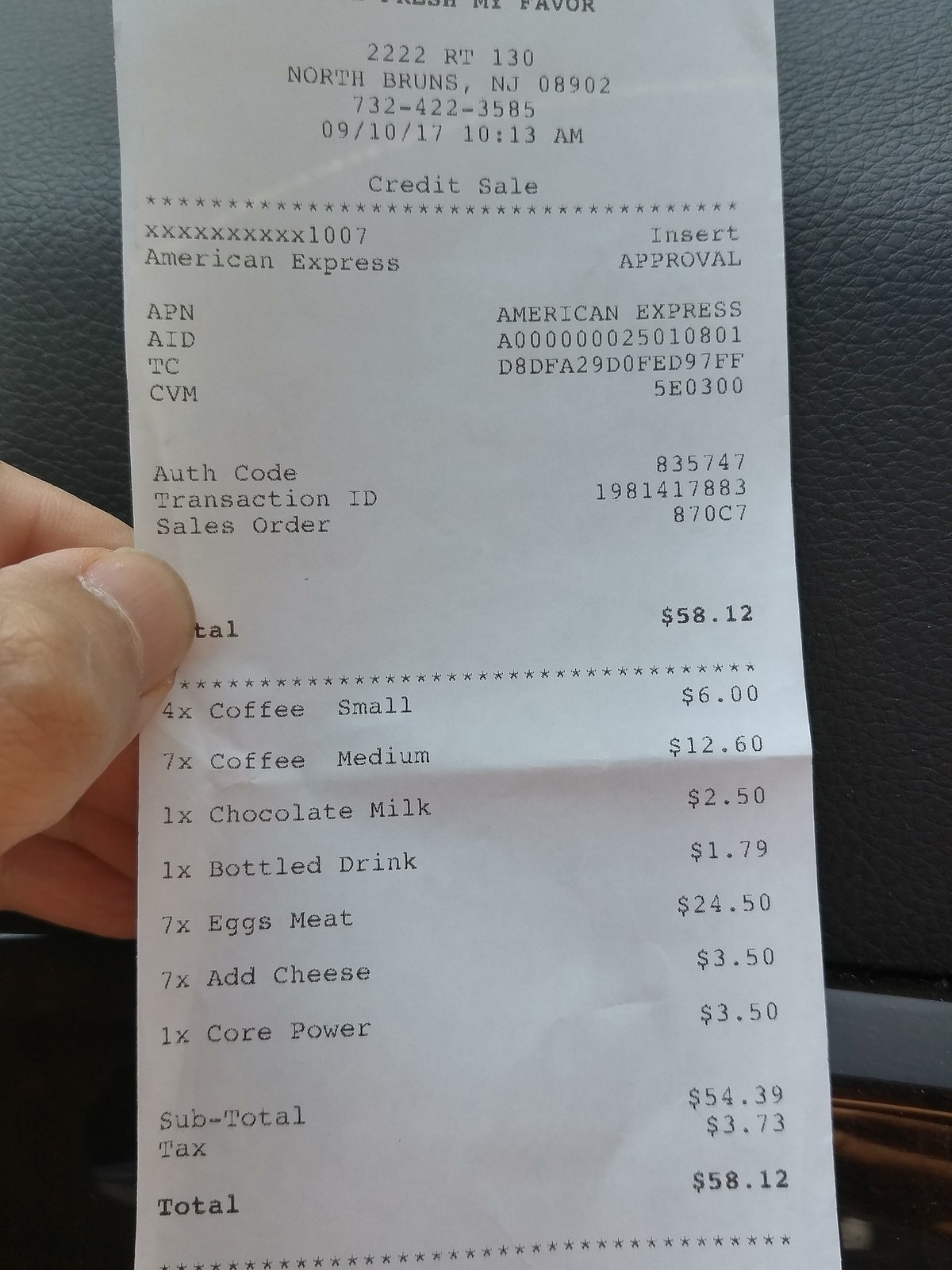This is a detailed photograph of a receipt being held by someone's hand inside a car, evident from the visible leather texture of the dashboard in the background. The photo, brightly lit by daylight, focuses primarily on the small, white receipt, which despite a central crease, remains crisp with unfaded ink. The receipt, dated 09-10-17 at 10:13 AM, is associated with an address and phone number: 2222RT130, North Bruins, New Jersey 08902, 732-422-3585. Though the retailer's name is partially visible, making out "favor" as part of it, the merchant details are mostly cut off. It's a credit transaction totaling $58.12, paid via American Express. The itemized purchases include four small coffees, seven medium coffees, one chocolate milk, one bottled drink, seven servings of "eggs, meat" (possibly sandwiches), seven "add cheese," and one CorePower drink. The sum of the items is noted as $54.39 with an added tax of $3.73, culminating in the final total.